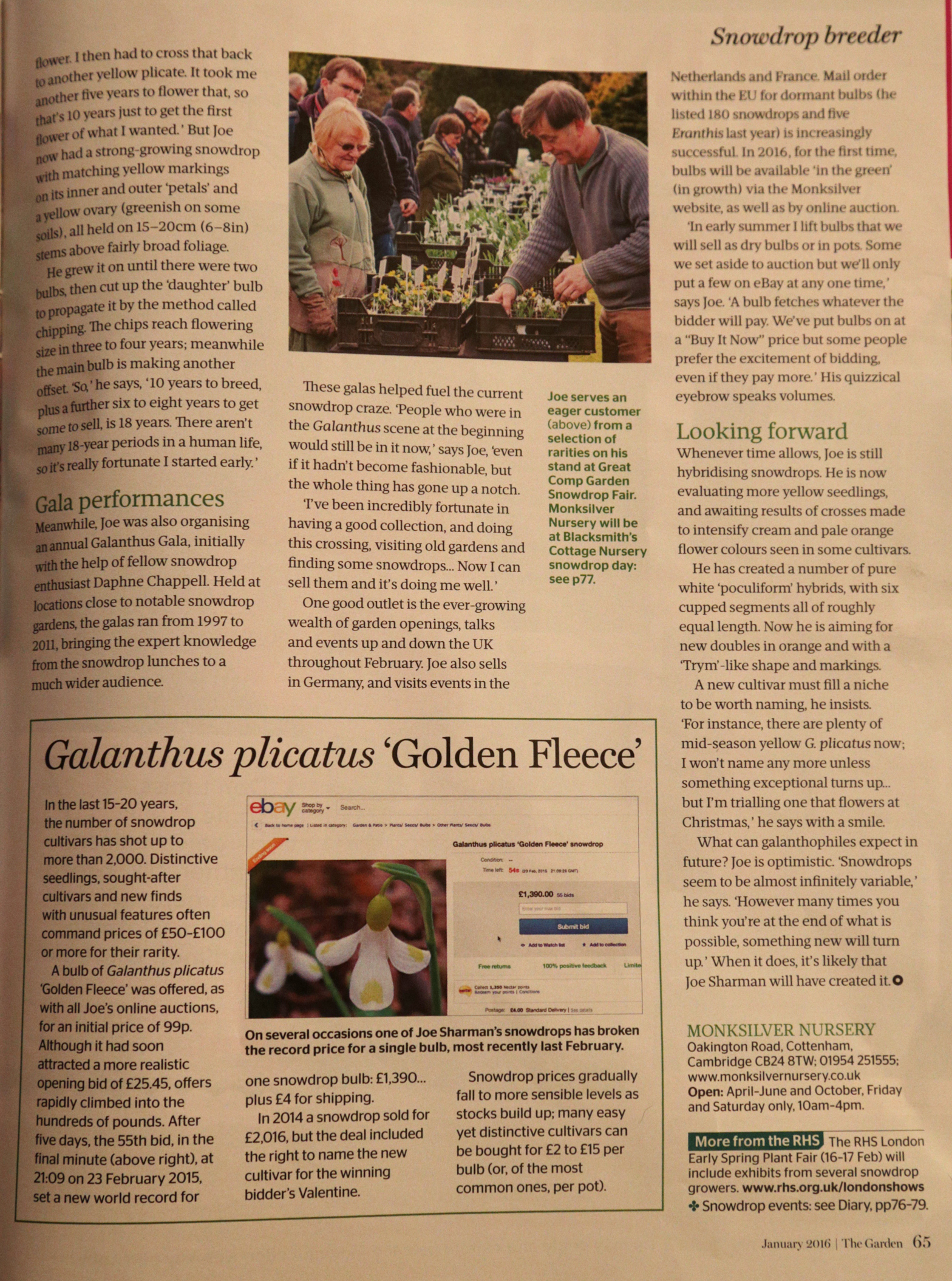This photograph captures an open book turned to page 65, as indicated by the page number in the bottom right corner. Adjacent to the page number, the text "January 2016 - The Garden" provides context for the content. The page is brimming with text that cannot be fully read due to the sheer volume, but several subheadings are visible, including "Gala Performances" and "Looking Forward." At the top of the page, a photograph features a group of individuals, ranging from middle-aged to elderly, examining crates filled with a variety of flowers. None of the flowers appear to be sunflowers, but they include various other colorful blooms. Towards the bottom of the page, a text box delivers additional information, mentioning terms like "gandalous," "placardus," and "golden fleece," with "golden fleece" highlighted in single quotes. Below this, there appears to be a second photo that likely depicts the flower mentioned in the text box, with a note suggesting it can be purchased on eBay. The page itself is predominantly white with black text, accented by touches of green and blue.